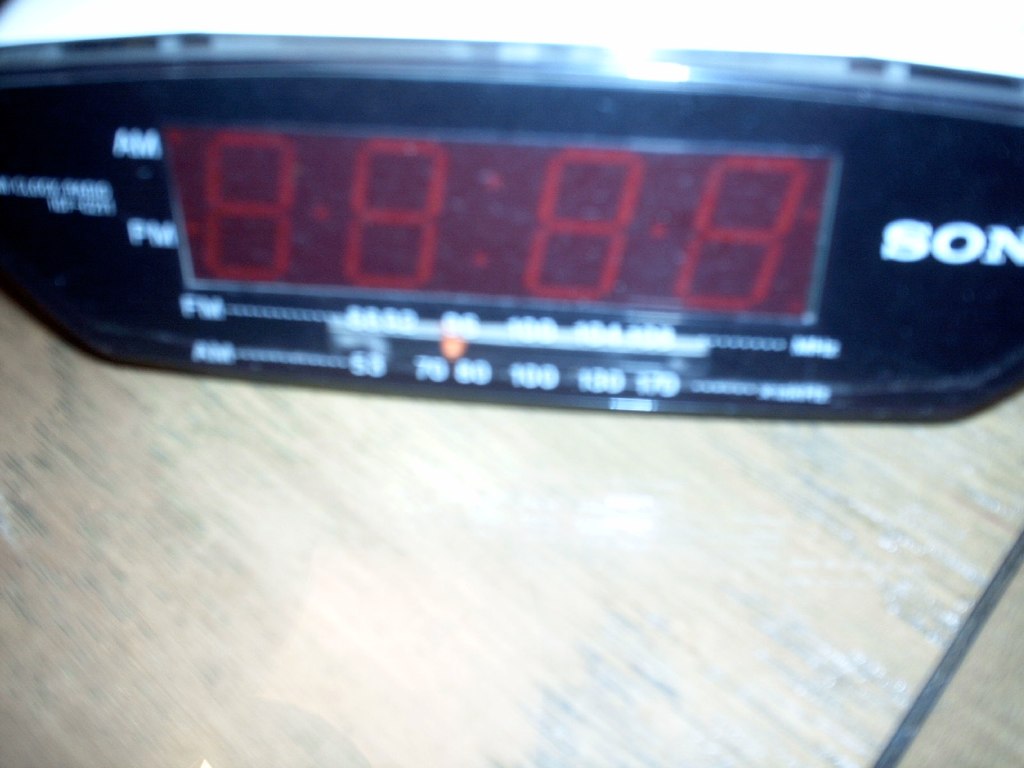The photograph captures an up-close, slightly out-of-focus image of a Sony digital alarm clock resting on a brown wooden table. The clock features a rectangular black body and a central digital display that currently shows a faint "8:88" with two colons in between, indicating that none of the numbers are lit. On the left side of the display, "AM" is written in white text above "PM." To the right of the display, the partial brand name "SON" is visible, signaling Sony. Below the display, there are sections for FM and AM radio frequencies, marked by a series of dots and numbers which are difficult to discern due to the blur. Notably, small orange dials are present for tuning the radio stations. The photo's low quality and close-up nature contribute to its slightly older and somewhat dated appearance.